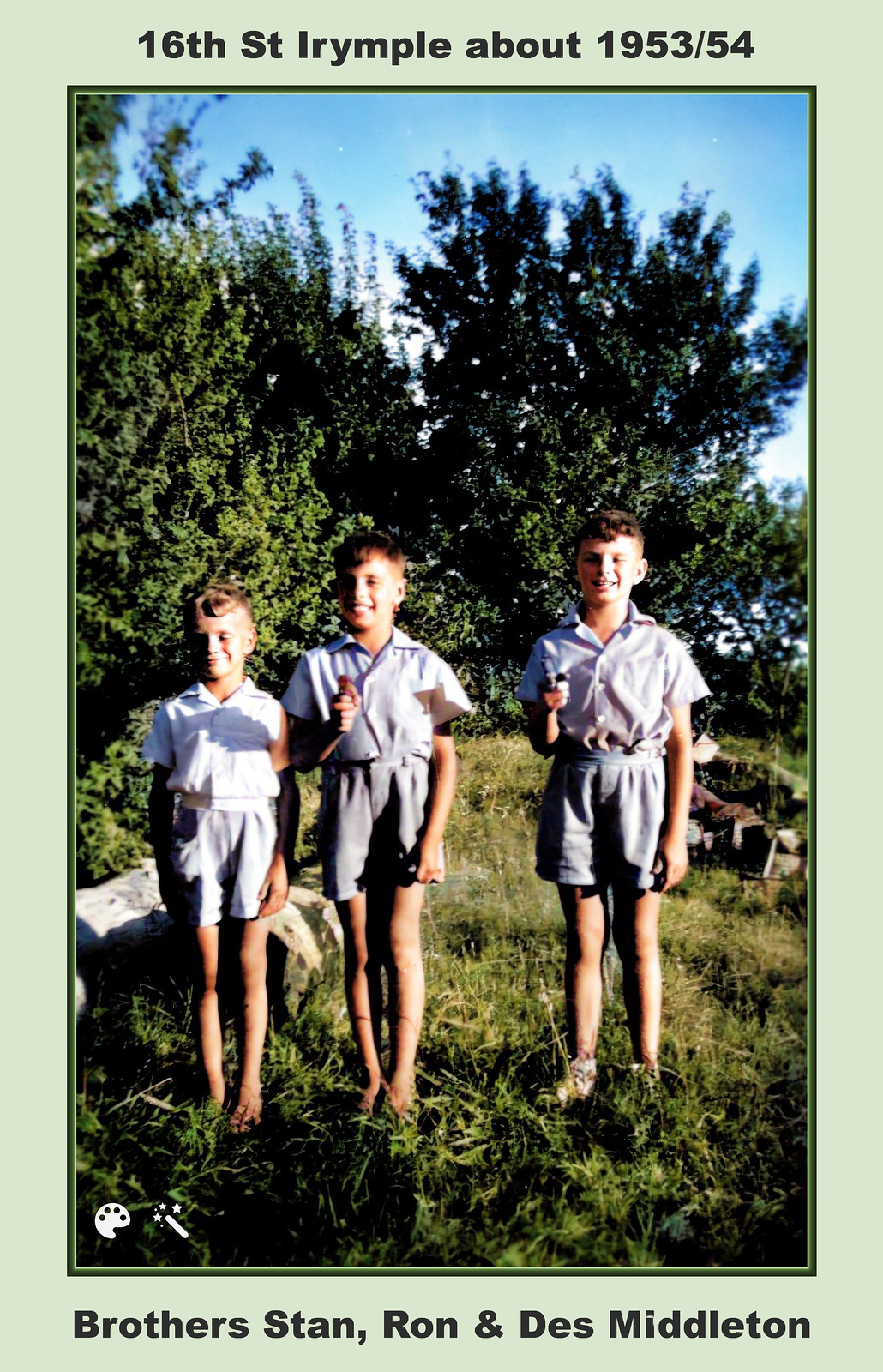This 1953-54 photograph captures three young boys, identified as Brothers Stan, Ron, and Des Middleton, standing outdoors in a grassy field. They are each dressed in matching outfits consisting of button-up collared shirts and shorts that go above their knees. Their cheerful smiles are evident as they pose amidst the greenery. The background showcases an array of very tall trees and some rocks, all under a clear blue sky devoid of clouds. The image is framed with a light green border, with the text "16th St. Arempel, about 1953-54" at the top and "Brothers Stan, Ron, and Des Middleton" at the bottom.